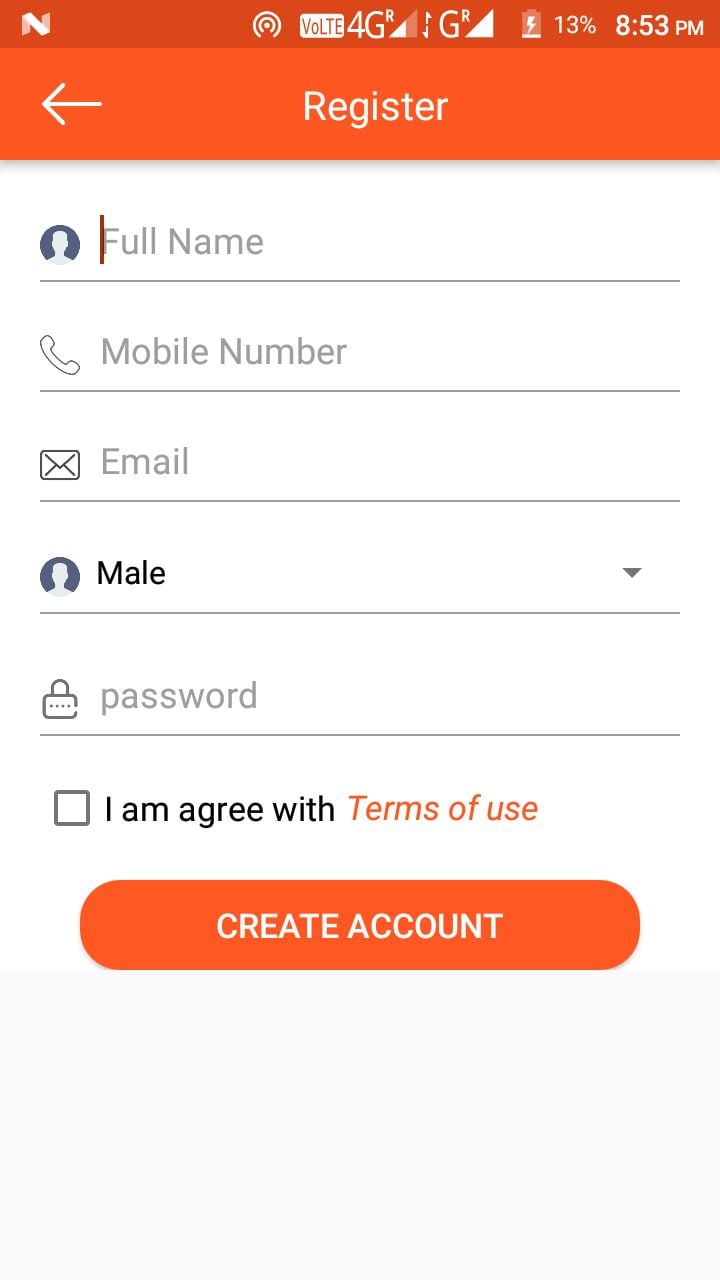In this image, a person is using a smartphone to create a new account. The smartphone appears to be a non-iPhone device, suggested by the unfamiliar button design. The screen displays several graphical elements in the top bar: a sideways "Z" logo, a concentric rainbow pattern forming an inward circle with decreasing radius lines, and a "VoLTE" (Voice over LTE) icon in a white box. Next to these, "4G" connectivity is indicated with a signal bar, showing half strength, and a network icon with a large "G" and small "R." A fully white box representing another network icon and a partially charged battery at 13% are also visible. The time reads 8:53 PM.

The main part of the screen shows a registration form. The form asks the user to enter their full name, phone number, and email address. Beneath these fields, there is a drop-down menu for selecting gender, with options for male and female. A password entry field follows, adjacent to a checkbox (currently unchecked) that says, "I agree with terms of use," where "terms of use" is an orange, clickable hyperlink. At the bottom of the form, there is an orange "Create Account" button with white text. There is also a back button allowing the user to return to the previous screen.